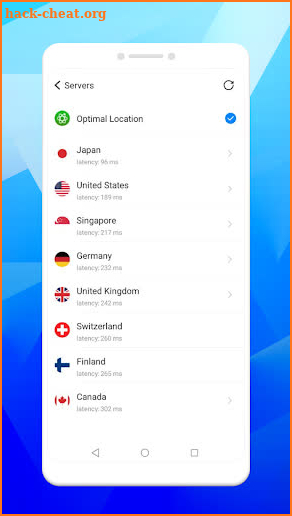Screenshot Analysis: A website screen from hack-cheat.org exhibiting server locations with a refresh button. Shows an 'optimal location' marked with a blue circle containing a white check. Available server locations include Japan, United States, Singapore, Germany, United Kingdom, Switzerland, Finland, and Canada, each with a right-pointing arrow. The background features a blue gradient, transitioning from dark at the bottom, resembling mountains, to light blue at the top. Bottom navigation icons include a left-pointing arrow, a circle, and a square, all set against a white background.